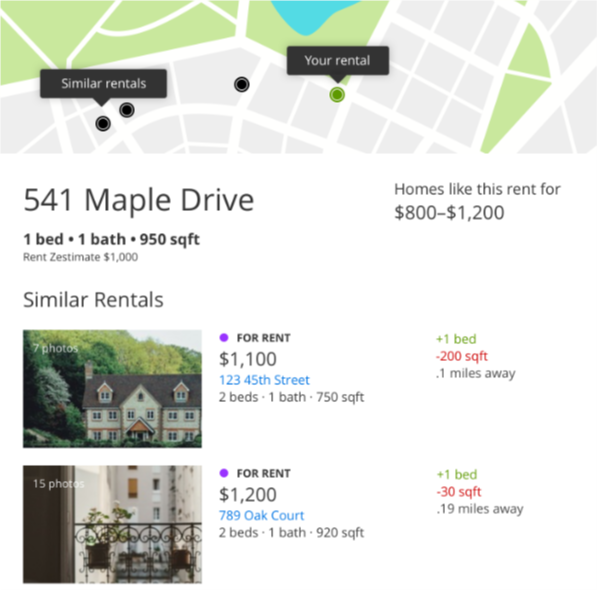**Detailed Caption:**

This is a screenshot from a real estate rental app, showcasing a simplified map graphic at the top section, which isn't imported data but rather a placeholder illustration. The map utilizes dotted black icons with speech bubbles; one indicates "similar rentals" and another identifies "your rental" marked in green.

Below the map, the main property highlighted is located at **541 Maple Drive**. To the left, in prominent text, it notes the address, while to the right it specifies that homes like this typically rent for **$800 to $1,200**. Detailed further, this particular listing features **one bedroom, one bathroom**, covering **900 square feet**. The estimated rent, termed as "Rent Zestimate," is set at **$1,000**, which might suggest the app could be associated with Zillow or a similar service, given the use of the "Zestimate" terminology.

Following this, there is a section entitled "Similar Rentals," displaying two results. 

1. The first option includes an image of a large, three-story house with a steep roof featuring **seven photos**. It's listed for **$1,100/month**, located at **1, 2, 3, 45th Street**. This option provides **two bedrooms, one bathroom**, and measures **750 square feet**, which is **200 square feet less** than the original property, positioned **0.1 miles away** from the initial listing.

2. The second option depicts a wrought iron balcony facing a set of vertical apartments or condos, possibly in a European style, with **15 photos** available. This property is listed for **$1,200/month**, located at **789 Oak Court**. It also offers **two bedrooms, one bathroom**, but is slightly larger than the first alternative with a size of **920 square feet**, **30 square feet less** than the primary property, situated **0.19 miles away** from the featured listing.

Overall, the presented data appears to be a mock-up, using dummy text to illustrate how the app might display similar rental options and their relative information.